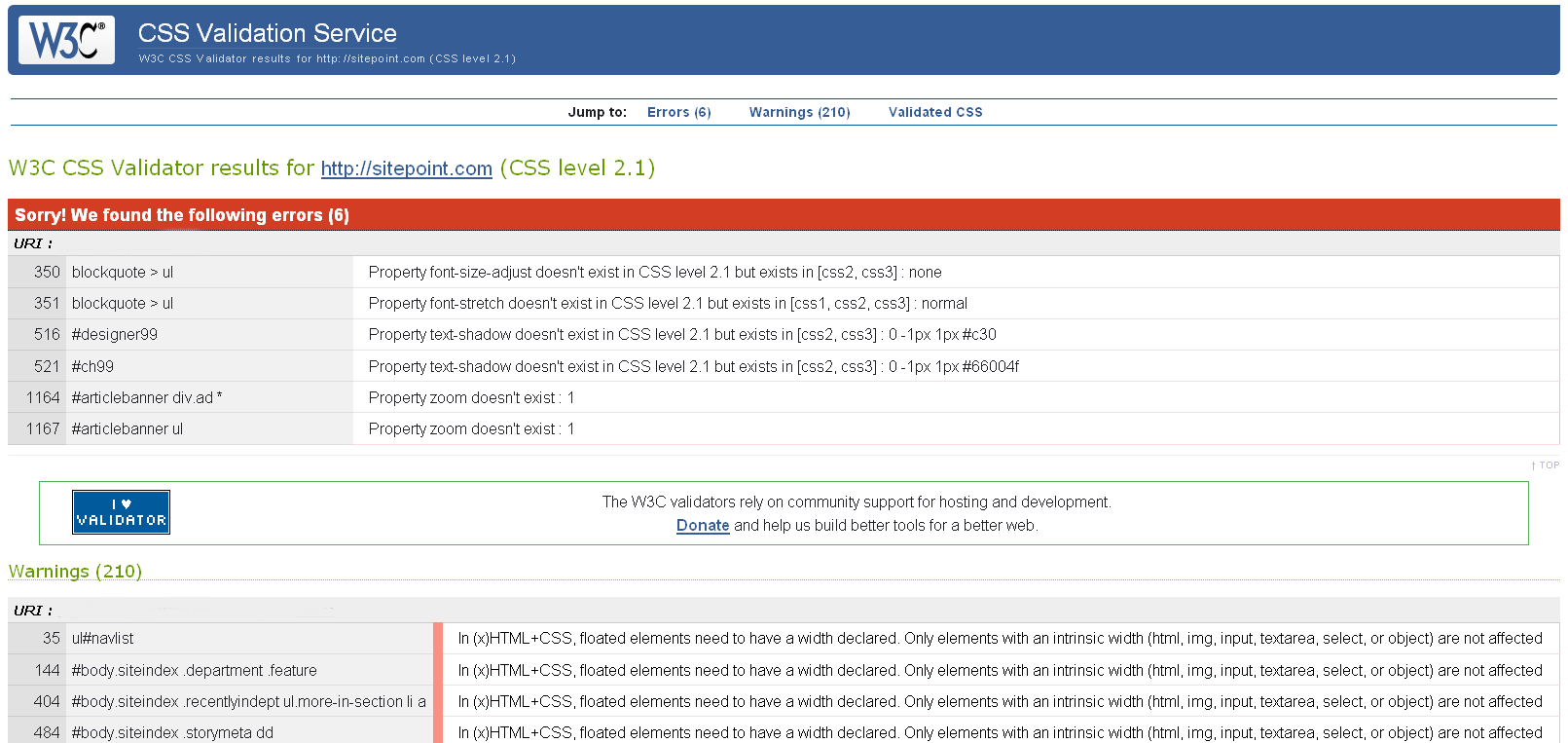The image displays a screenshot of the CSS Validation Service provided by W3C. The W3C logo is featured, with the 'W' in a distinct blue color and the 'C' in white. The validation service has options such as "Jump to Errors" with an indication of six errors in parentheses, "Warnings" followed by a count of 210 in parentheses, and a section titled "Validated CSS" with W3C and CSS Validated Results. The results appear highlighted in green.

The main body of the page features a hyperlink styled in blue that directs to http://sitepoint.com, annotated with "CSS Level 2.1" in green parentheses. A red rectangle with white text alerts, "Sorry, we found the following errors (6)," indicating there are six errors to address. Each error is listed with a specific number and description, including error codes like 350, possibly 301 or 351, 516, 521, 1164, and 1167.

Additionally, a blue rectangle with white letters displays the message "I Love Validator." Below the error section, a warning list signifies there are 210 warnings, presumably detailed in an extensive list.